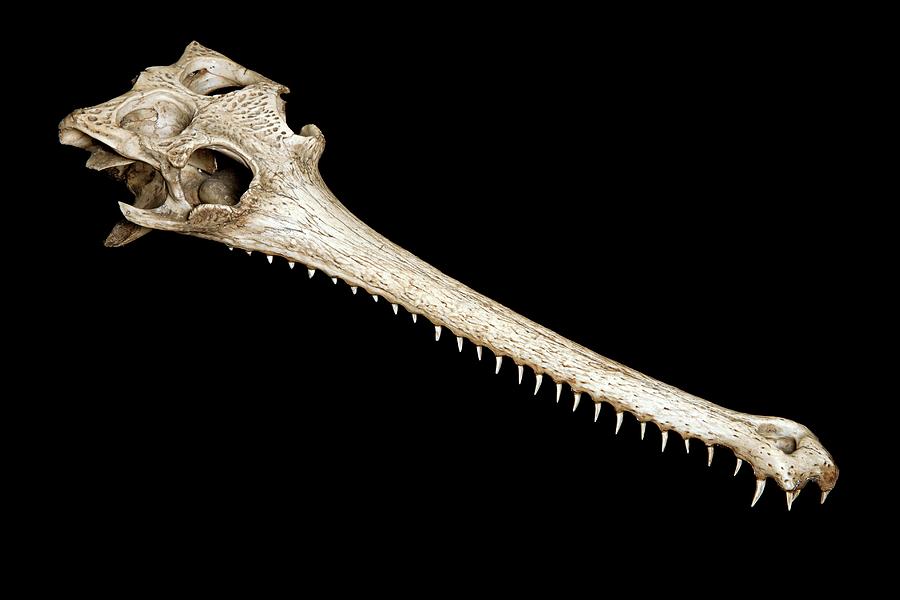The image is a detailed photograph of an elongated animal skull, potentially that of a gharial or a similar species like a crocodile. The skull, light tan in color, prominently features a remarkably long snout that is approximately five to six times the length of the cranial portion. The numerous teeth protruding from the snout are sharp and cone-shaped, with the teeth near the front being longer and more pointed compared to the smaller, duller ones towards the back. Notably, only the upper jaw is visible, lacking a bottom jaw. Positioned diagonally across the image, the broader cranial base is at the top left, tapering down to the narrow snout at the bottom right. Eye sockets and large cavities near the base of the skull are clearly visible, along with various imperfections, lines, and pitting that add to the skull’s textured appearance. The entire skull is set against a completely solid black background, emphasizing its intricate details.